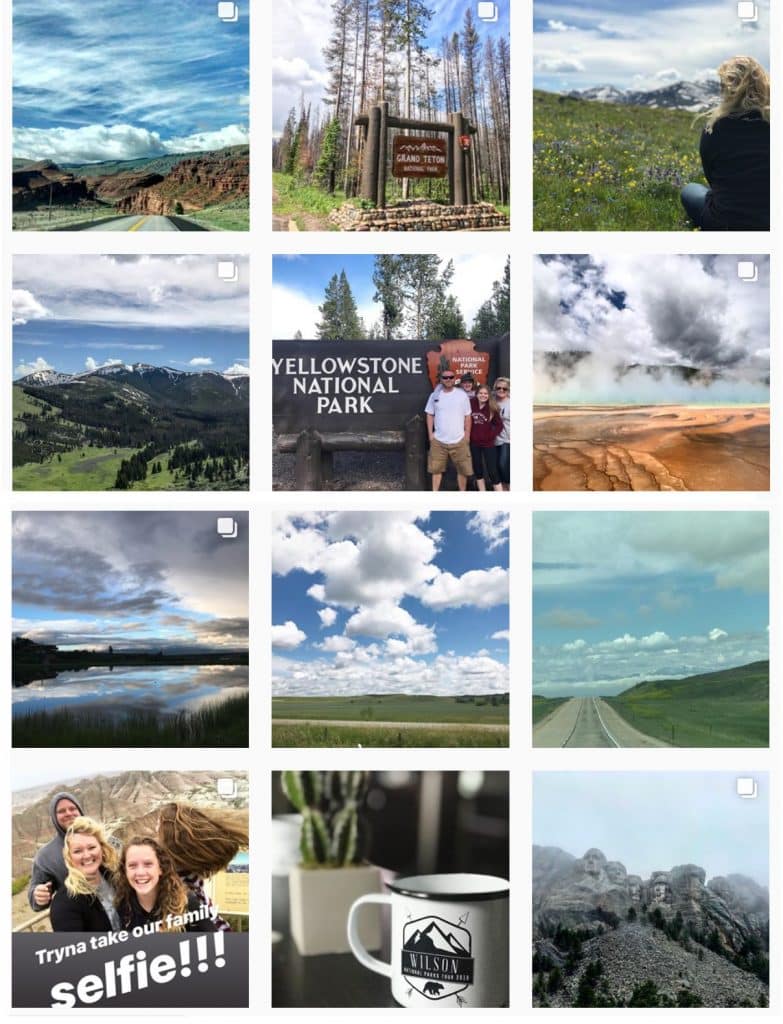This image captures a snapshot of an Instagram profile page displaying a grid of 12 photos. There is no visible title or username, but the familiar Instagram layout is unmistakable. Each photo showcases different scenes from a vacation, predominantly featuring breathtaking landscapes and moments from Yellowstone National Park. In three of the photos, a family—comprised of a man, a woman, and two younger individuals presumed to be their children—pose together, with one image specifically highlighting their visit to the Yellowstone National Park sign. The remaining nine photos beautifully depict the natural splendor of Yellowstone, including majestic mountains, towering trees, expansive skylines, and an inviting scene inside a cozy coffee shop.